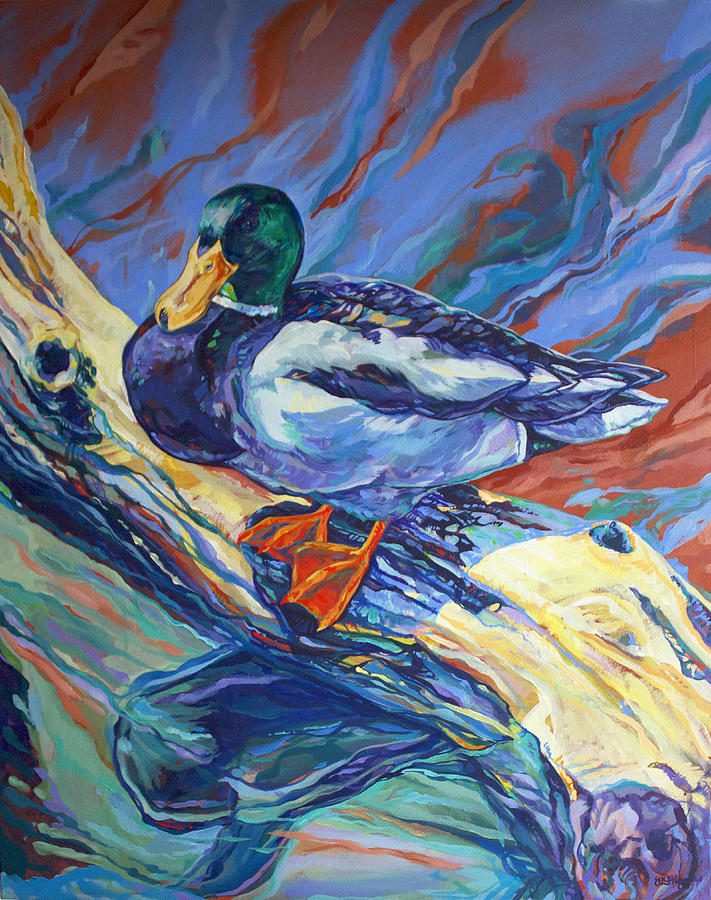The image portrays a vibrant, modern watercolor-style jigsaw puzzle featuring a solitary mallard duck at its center. The mallard stands confidently on a log, which is artistically rendered in shades of white, yellow, and orange. Beneath the duck's tail, its shadow adds depth to the scene. The duck's orange feet grip the log firmly as it gazes forward, showcasing a dark blue breast and light blue undertail feathers. The upper feathers vary between dark blue and lighter hues, while its head is a distinctive green, typical of a mallard, with a striking yellow bill.

The background bursts with color, primarily swirling blue hues accented with streaks of orange and green, creating an almost fiery effect. These painterly strokes contrast beautifully against the detailed depiction of the duck. Below the log, a shimmering lake reflects the duck in deeper blue tones. The water itself is a dynamic mixture of greens and pinks, giving the illusion of movement, as if flowing.

Further enhancing the scene, the area behind the duck contains ambiguous orange blobs, possibly suggesting fish swimming beneath the water's surface. The overall composition cleverly blurs the distinction between sky and water, enhancing the surreal and mesmerizing quality of this modern jigsaw puzzle artwork.